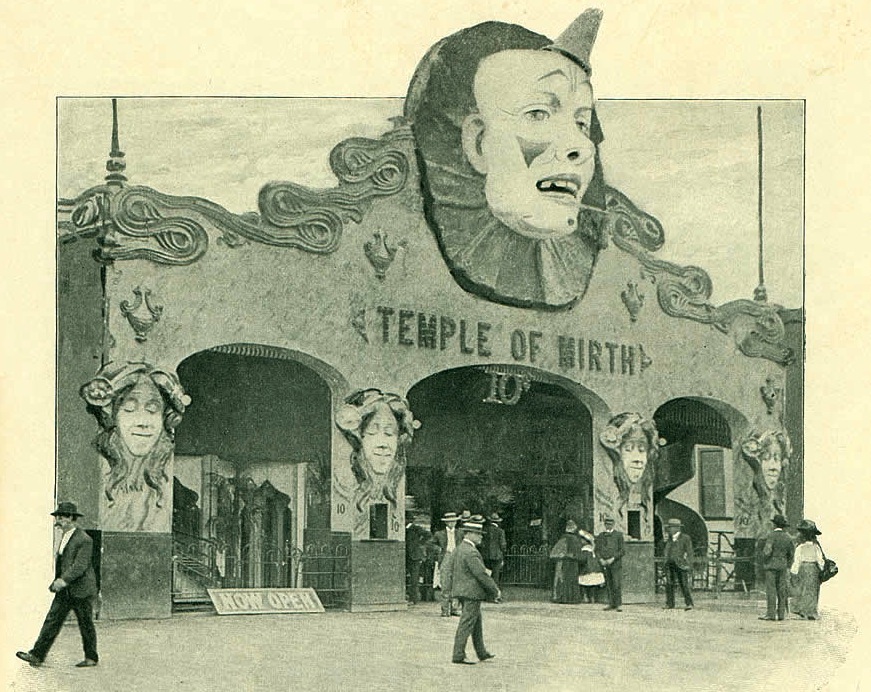The image is a landscape-oriented, black and white photograph from what appears to be the early 20th century, likely the 1920s or earlier. The scene captures the entrance to a building labeled "Temple of Mirth" in large, capitalized letters above the central arch of three grand arches that dominate the facade. A large, exaggerated clown face with a tiny hat, big neck ruffle, and triangular makeup adorns the area above the Temple of Mirth sign, with ribbon-like decorations extending from its sides. Below the sign, a smaller inscription indicates an entrance fee, stating "10 cents."

The structure is adorned with intricate carvings, including the faces of women with closed eyes and flowers in their hair, placed between the arches as if they are supporting the building. A "Now Open" sign is prominently displayed at the bottom left corner of the entrance.

The photograph, possibly a scanned image, features a slightly stylized off-white border around a starkly contrasted, clear image. The background reveals a clear sky with ample daylight illuminating the scene. In the foreground, men and women dressed in period-specific attire, including flat straw hats, round bowler types, long sleeves, and dresses with hats, are seen walking in and out of the building. The overall composition captures a bustling moment at this whimsical, carnival-like venue, providing a nostalgic glimpse into a bygone era.